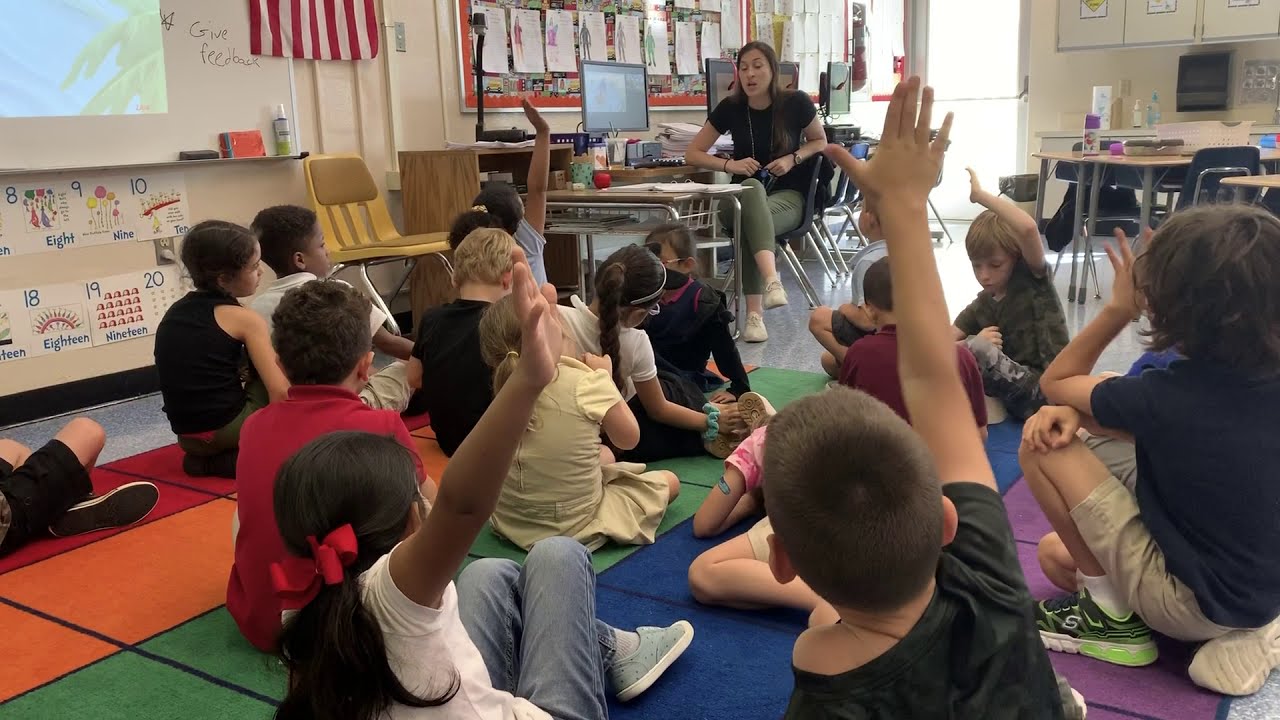In this captivating photograph, a classroom setting comes to life with vibrant details. The scene showcases a dedicated teacher, likely in her early 30s, with black hair and clad in a black t-shirt, green pants, and white tennis shoes, engaging with a group of eager young students. She is seated at a desk with a computer monitor to her left, positioned against a backdrop featuring a lively display of children's drawings and an American flag. Surrounding her, the walls are adorned with educational aids, including a series of numbered prints (8, 9, 10, 18, and 19) hinting at kindergarten activities.

The children, who appear to be in kindergarten or first grade, are seated on a soft, colorful mat composed of square tiles in shades of orange, red, green, blue, and purple. The majority of the children are dressed in black shirts and khaki shorts, though a few standout outfits catch the eye—a girl in a brown dress, another in a white shirt and jeans, and one in a yellow dress with blue jeans and blue tennis shoes. 

Several students have raised their hands, eagerly participating in the lesson. To the right of the teacher is a table topped with what might be a monitor or a microwave, surrounded by containers and chairs. The ambiance is further enriched by light streaming through a door in the background, contributing to the inviting atmosphere of this educational space.